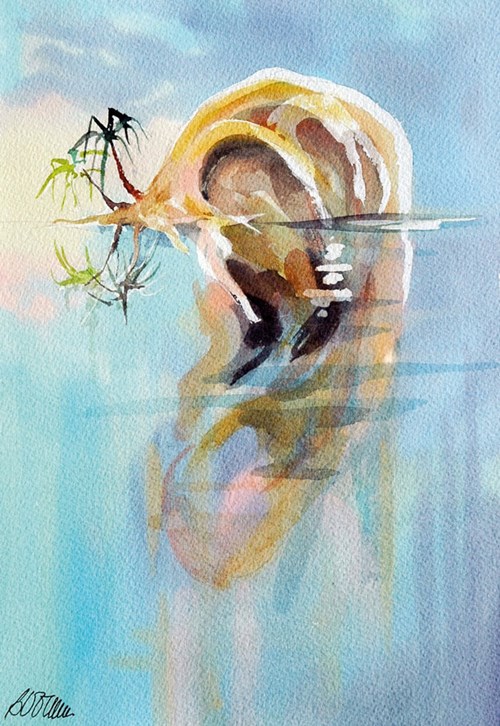The image is a vivid watercolor painting featuring a small island surrounded by a body of water. Dominated by shades of blue, with touches of pink and purple where the colors blend, the scene evokes a tranquil, almost whimsical atmosphere. At the center of the composition is an island that resembles an earlobe in shape, descending underwater, accentuated with a yellow hue and subtle black and brown shading topped with white highlights, giving it a textured and three-dimensional feel. 

Above the island, the sky is a bright, natural blue with soft clouds and a hint of sunlight on the top left corner, adding brightness and warmth to the scene. Two palm trees stand on the left side of the island, one with dark green leaves and the other with lighter green, both leaning slightly towards the water, their reflections elegantly mirrored on the water’s surface. 

The overall composition is completed with a signature in the bottom left corner, although it's faint and hard to decipher. The natural lighting and clear setting of the painting make it a captivating, serene portrayal of a tropical oasis.